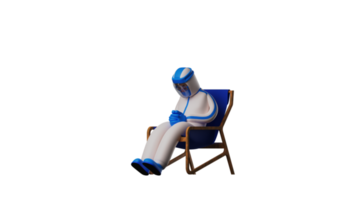The image depicts a cartoon figure dressed in a white full-body suit featuring a blue stripe that runs down the center from the neck, branching into the arms and covering the hands. Blue gloves and blue shoes complement the suit, and the face is covered by a blue helmet with an oval shape over the face, adorned with lines extending like a crown—one line stretches from the center of the head to the back, and another wraps around the head like a headband. The figure is seated in a simple-framed chair that appears to be wooden or metal, with a darker blue cloth seat, distinct from the blues found on the suit. The chair is slightly reclined, and the figure looks disengaged, possibly sleeping or resting with their head tilted downwards.